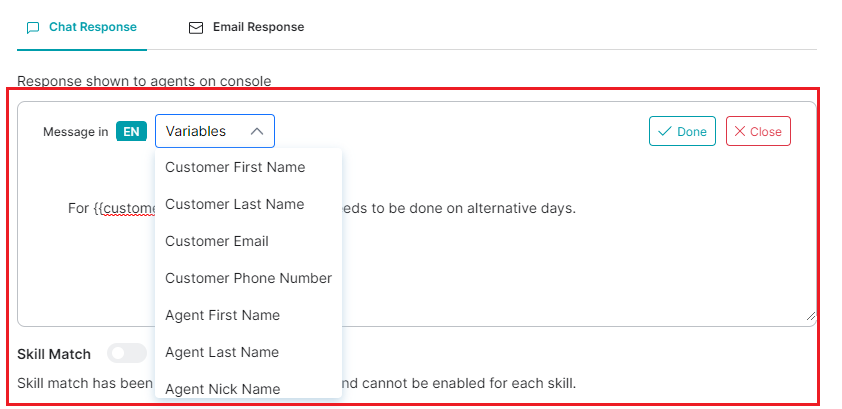The image depicts a user interface with a prominent red-lined box highlighting a specific section. Within this section, there is a smaller, whiter box. This inner box contains various elements crucial to the interface's functionality:

- In the upper left-hand corner of the whiter box, there is a message area.
- Adjacent to the message area, there is a greenish box with the text "EN" in white font, indicating the language setting as English.
- Next to the language setting box, there is a dropdown menu labeled "Variables." When expanded, this menu reveals several options, including:
  - Customer First Name
  - Customer Last Name
  - Customer Email
  - Customer Phone Number
  - Agent First Name
  - Agent Last Name
  - Agent Nickname

Additionally, in the upper right-hand corner of the whiter box, there are two buttons labeled "Done" and "Close," allowing the user to finalize their actions or exit the interface, respectively. The image provides a detailed snapshot of the interface designed for user interaction and data entry by agents on a console.